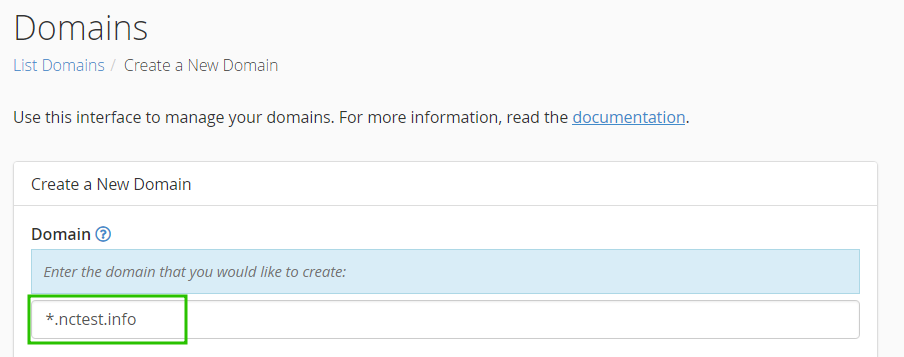**Descriptive Caption: Screenshot of Domain Management Interface**

The image is a screenshot of a domain management window. At the top left corner, the header reads "Domains." Directly beneath this header, there is a blue text link labeled "List Domains / Create a New Domain." Here, "List Domains" is in blue, indicating it as a clickable link, while "Create a New Domain" is in black.

A small section separates the header from the next line, which instructs: "Use this interface to manage your domains. For more information read the documentation." The word "documentation" is hyperlinked and underlined, suggesting it provides additional resources.

Below this instructional text is a white chart titled "Create a New Domain." The body of this chart begins with the label "Domain" accompanied by a blue question mark icon, likely offering help or additional information.

Underneath, a blue banner with italicized text instructs users to "Enter the domain that you would like to create." Below this banner is an input bar for entering domain information. Part of the bar is highlighted within a green box that contains the text "* .nctest.info," serving as an example or placeholder. The chart or box's overall background is white, while the broader domain section has a subtle light gray shade to distinguish it.